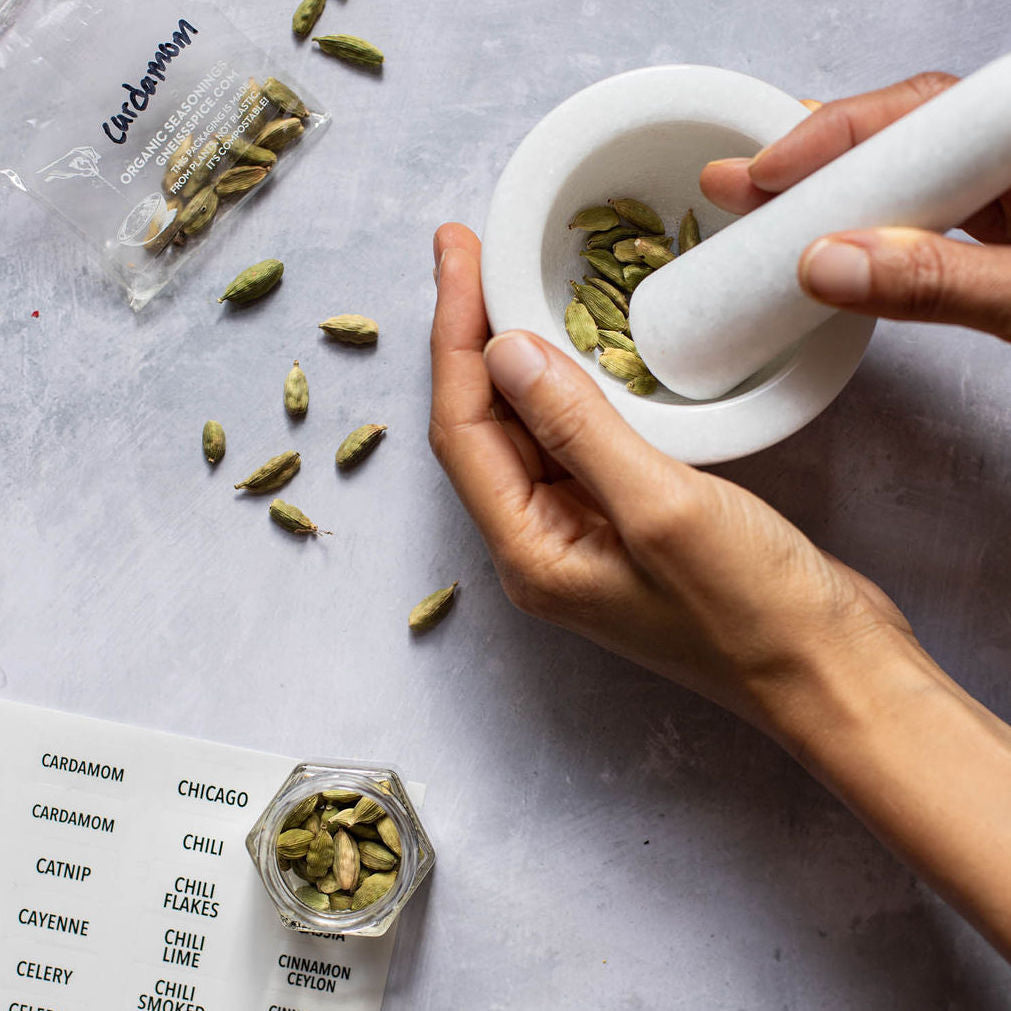An indoor, close-up color photograph of a person using a mortar and pestle to grind cardamom seeds on a light gray, slate-colored counter. The person's light-skinned left hand, extending in from the right edge of the image, is steadying a white, likely marble, mortar, while their right hand is holding the pestle, poised to grind the seeds within. Scattered around the white mortar are several light green, oval-shaped cardamom seeds. In the upper left corner of the image, a clear plastic bag, labeled in black Sharpie as "cardamom" and printed with "organic seasoning" from chensingpiece.com, is visible. Below it, in the lower left corner, a glass jar filled with more cardamom seeds sits on top of a white sheet featuring labels for various seasonings such as cardamom, cayenne, catnip, chili, chili flakes, chili lime, and cinnamon. A few seeds are also seen scattered on the table, adding to the rustic and detailed atmosphere of the scene.